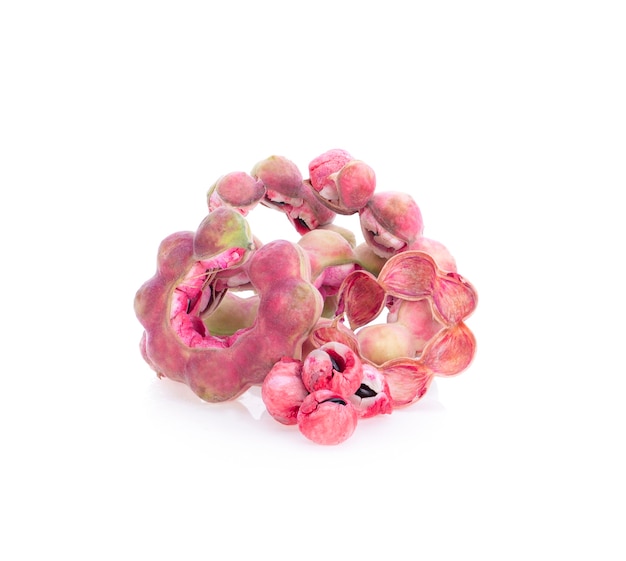The photograph showcases a tightly clustered arrangement of berries, predominantly in shades of pink and red, with occasional hints of green around the edges. The berries are of uniform size, roughly that of a grape, and some appear to be slightly open, revealing dark centers that might be pits or a type of gel. Prominently on the right side, a circular formation resembling a donut is visible, adorned with smaller, cherry-like berries. These berries exhibit a textured surface, with some forming intricate, intestine-like patterns winding through the cluster. Amidst the predominantly pink and red hues, a single berry stands out with its pale yellow color, tinged with pink. The specific type of plant these berries belong to remains unidentified, and details such as edibility or plant origin are not provided within the context of the image.